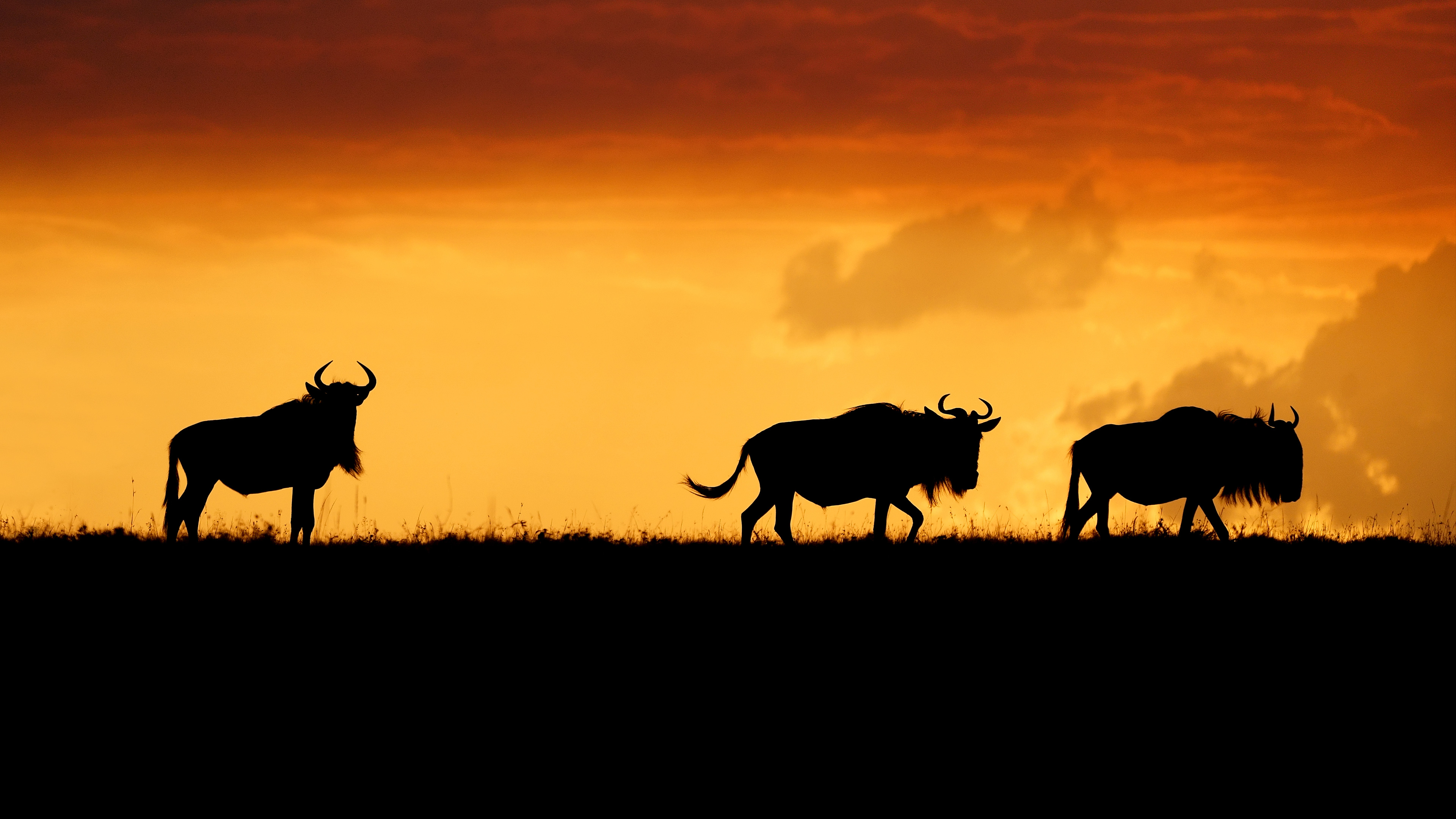In this captivating photograph taken outdoors at either dawn or dusk, three silhouetted wildebeests grace the horizon, walking atop a hill on a savanna or open prairie, likely in Africa. The image showcases their distinct outlines and cow-like forms, complete with four legs, two horns, and long tails. The composition is framed with the sun setting in the background, casting a stunning gradient across the sky—from a golden-yellow at the bottom to deep orange and reddish tones at the top. The sky is interspersed with some clouds, their tops tinged with reddish hues reflecting the sunlight. The dark, spiky grass at the hill’s edge contrasts sharply with the vivid sky, creating a stark yet beautiful silhouette. The arrangement captures two wildebeests walking in front of the third, which stands slightly apart and gazes directly at the camera, adding a moment of connection in this breathtaking landscape.